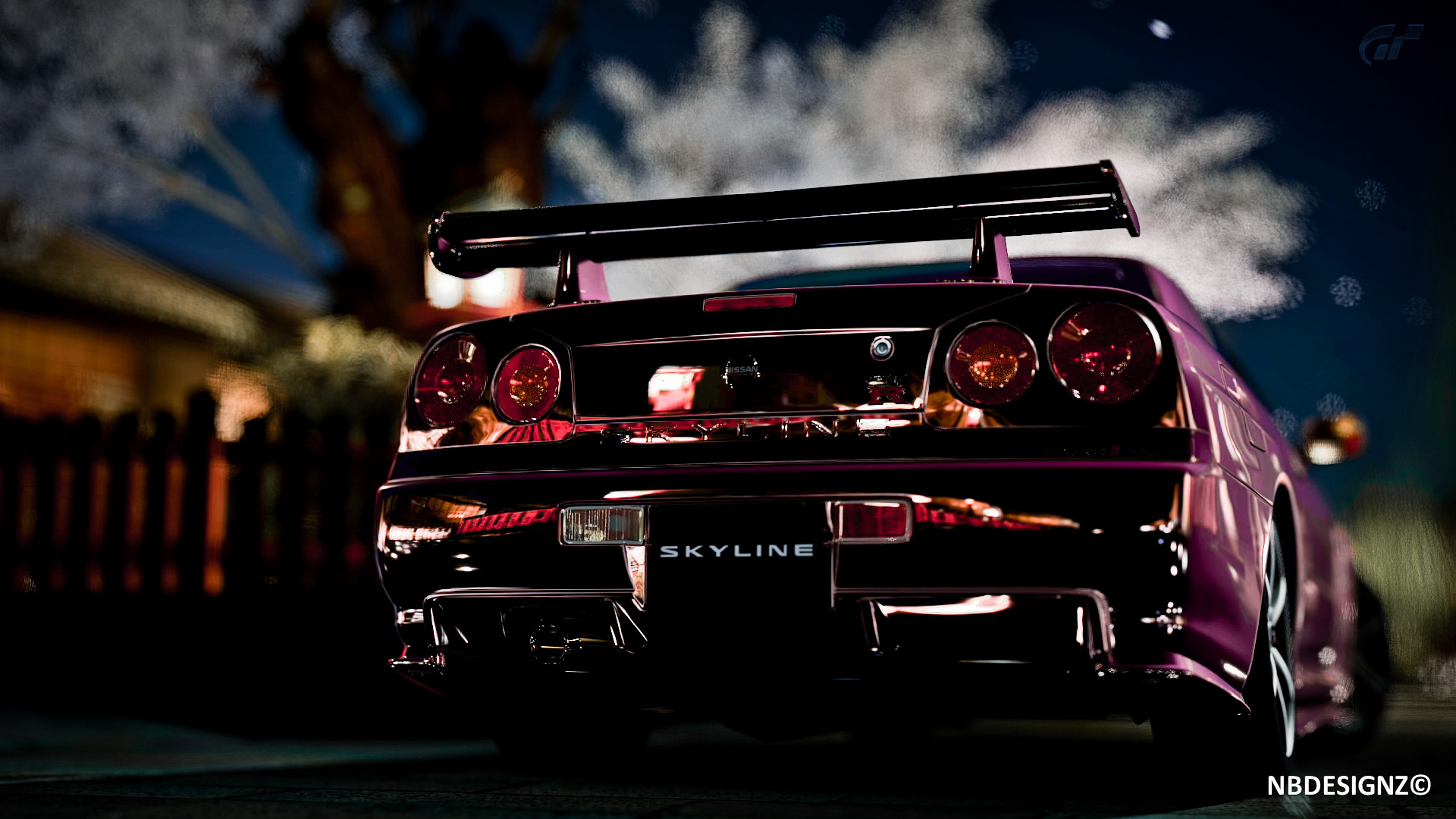The image is a stylized, dramatic color photograph showcasing the rear end of a brand new, deep purple sports car, specifically a GTR Nissan Skyline. The car is featured in an advertisement, and its back license plate area prominently displays the word "SKYLINE" in white capital letters on a black background. The car includes a prominent spoiler, tail lights, and brake lights. In the lower right corner of the image, the text "NBD DESIGNS" with a Z in copyright is visible in white.

The background of the image is slightly blurred, with a dark blue night sky and silhouettes of trees. On the left side, there is a wooden picket fence in front of a house. The dramatic filter effect applied to the image enhances the colors, making them pop significantly. No individuals or specific location details are present in the advertisement.